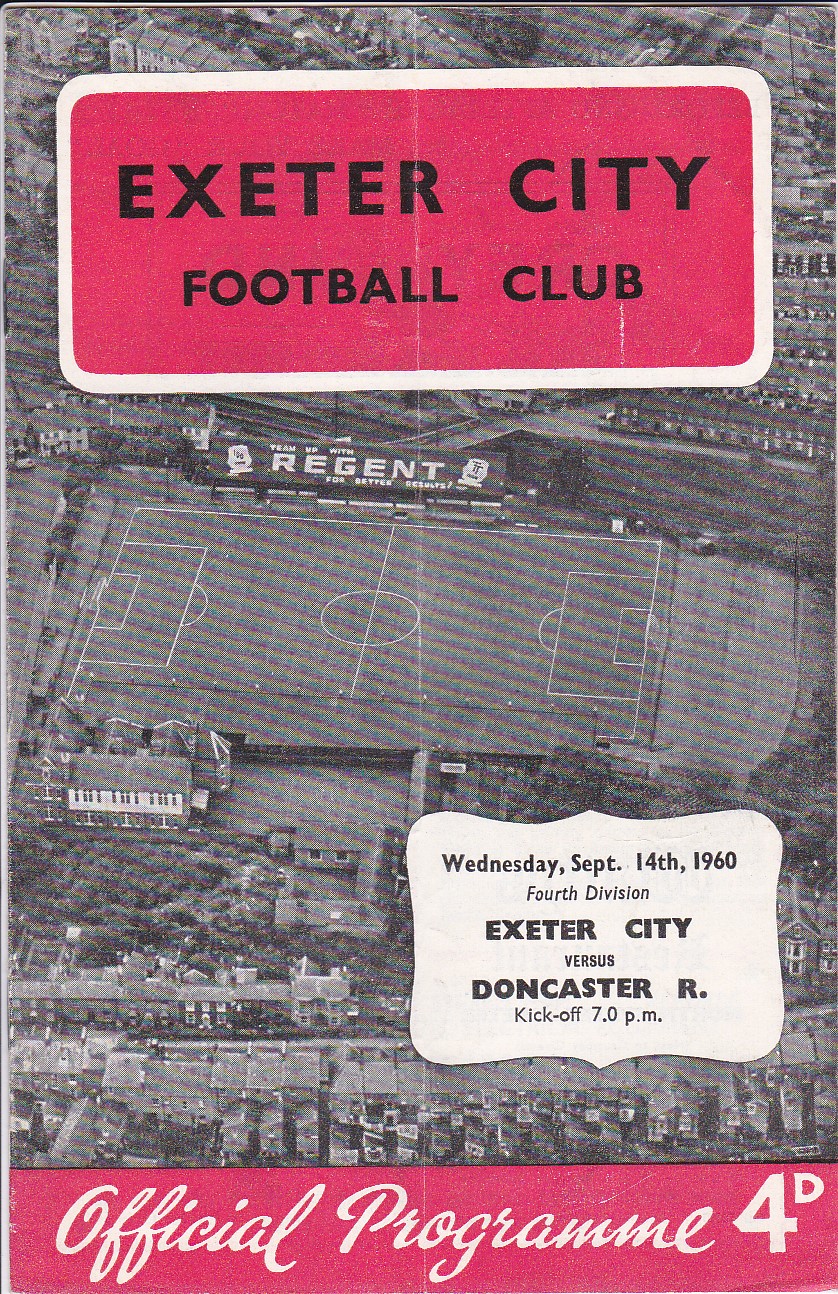The cover of this vintage soccer program from Exeter City Football Club features a gray and pink color scheme. At the top, it prominently displays "Exeter City Football Club" in black letters on a pink background. Beneath this title, there is an aerial, black-and-white photograph of a soccer field, emphasizing its historical aspect. The program informs about an upcoming 4th Division match: "Wednesday, September 14, 1960, Exeter City vs. Doncaster R, kickoff 7 p.m." This text is set within a decorative rectangle on the lower right corner of the image. At the very bottom, it states "Official Program 4D" in white script on a pink background, solidifying its purpose as a matchday program.